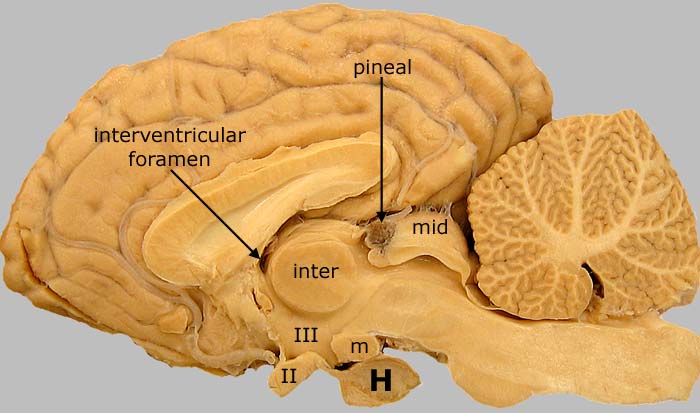This image features a highly detailed side view model of a human brain. The model is rendered in a light orange or tan color, showcasing the intricate wavy ridges characteristic of the human brain's texture. It displays a cross-section of the brain, focusing on one hemisphere, allowing a clear view of the internal structure. Several parts of the brain in this model are marked and labeled with black arrows and text. Notable labels include the "interventricular foramen" and the "pineal gland". Additional text labels identify regions with terms such as "mid" and "inter", as well as Roman numerals "II" and "III". Letters such as "M" and "H" also mark specific areas. The background of the image is grey, providing a neutral backdrop that emphasizes the detailed anatomical features of the brain model.